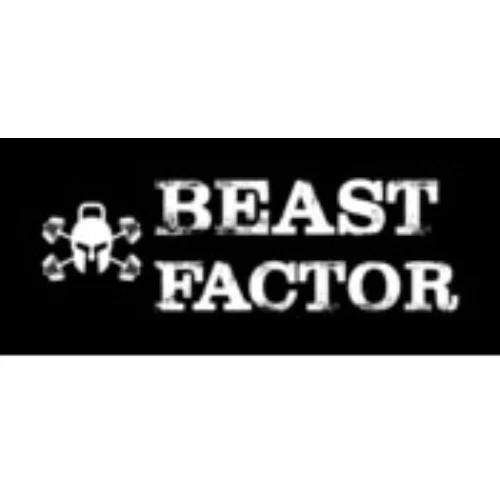This rectangle-shaped image, reminiscent of a horizontal TV or theater screen, features a solid black background. Dominating the center-right portion are two lines of text in large, white block letters, which appear worn and distressed with black showing through. The top line reads "BEAST," while directly under it, in slightly smaller but equally bold font, the word "FACTOR" is perfectly aligned to match the width of "BEAST."

On the left side of the image is an intriguing graphic: a helmet-like mask that conveys a sense of toughness or warrior-like strength. This mask has four protrusions that resemble stylized weapons or possibly dumbbells, resembling something akin to a skull and crossbones design. Moreover, the helmet features a handle, making it look similar to a kettlebell, suggesting themes related to fitness or exercise. The overall composition and imagery suggest that it could be related to fitness branding or advertising.